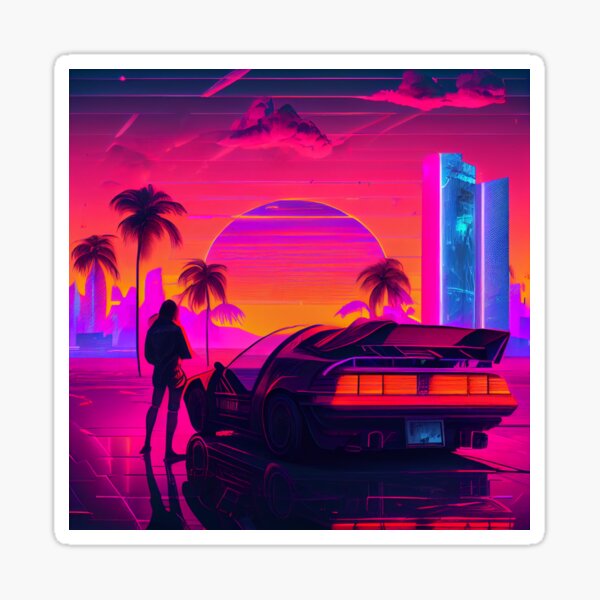The image is a vibrant, square piece of vaporwave artwork, boasting a thick light gray border that presumably represents the wall it hangs on. The artwork itself is square with rounded corners, accentuated by a thin white border. The composition exudes a distinctive 80s synthwave aesthetic, emphasizing neon colors like pink, purple, blue, and orange. Central to the piece is a woman standing next to a futuristic car that resembles a DeLorean or Trans Am, with the car displaying glowing red taillights and a large spoiler, both standing out against the neon-pink, shiny ground. In the background, a neon-colored sunset blends hues of purple, pink, orange, and yellow, setting the tone for the entire image. Silhouetted palm trees and glowing skyscrapers, rendered in vivid blue and purple, populate the midground. A grid pattern overlays the ground, sun, and sky, enhancing the retro-futuristic vibe.